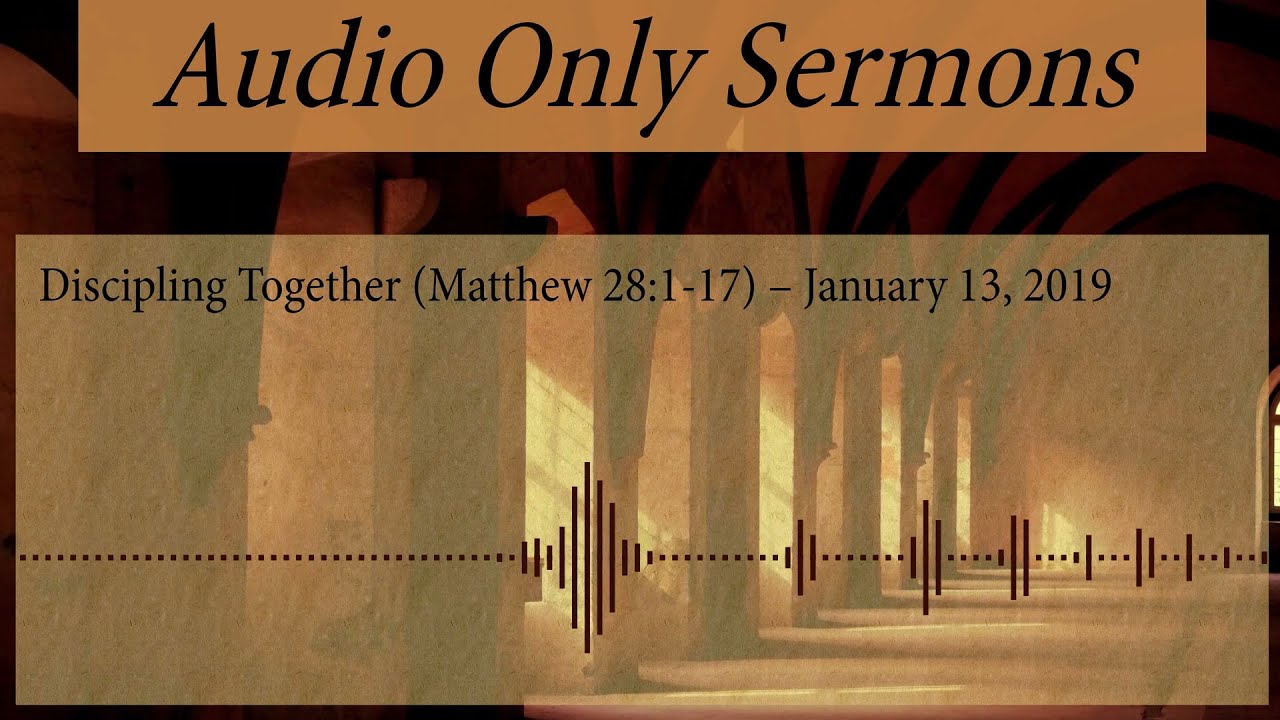This horizontal rectangular graphic resembles an informational card featuring a predominantly text-centric design. At the top, there's an orangish-brown rectangle with the phrase "Audio Only Sermons" inscribed in black. Below, there's a larger, lighter brown rectangle occupying the middle to the bottom of the image. This section reads "Discipling Together (Matthew 28:1-17) - January 13, 2019" in black text. A dark brown dashed line adorns the bottom of this large rectangle, resembling sound wave patterns with alternating dots and vertical lines, akin to audio signal visuals.

The background displays a dark brown architectural scene, featuring a grand arched ceiling and tall stone columns, giving the impression of an old church or similar structure. The entire composition has an orange-brown hue that ties the elements together cohesively.